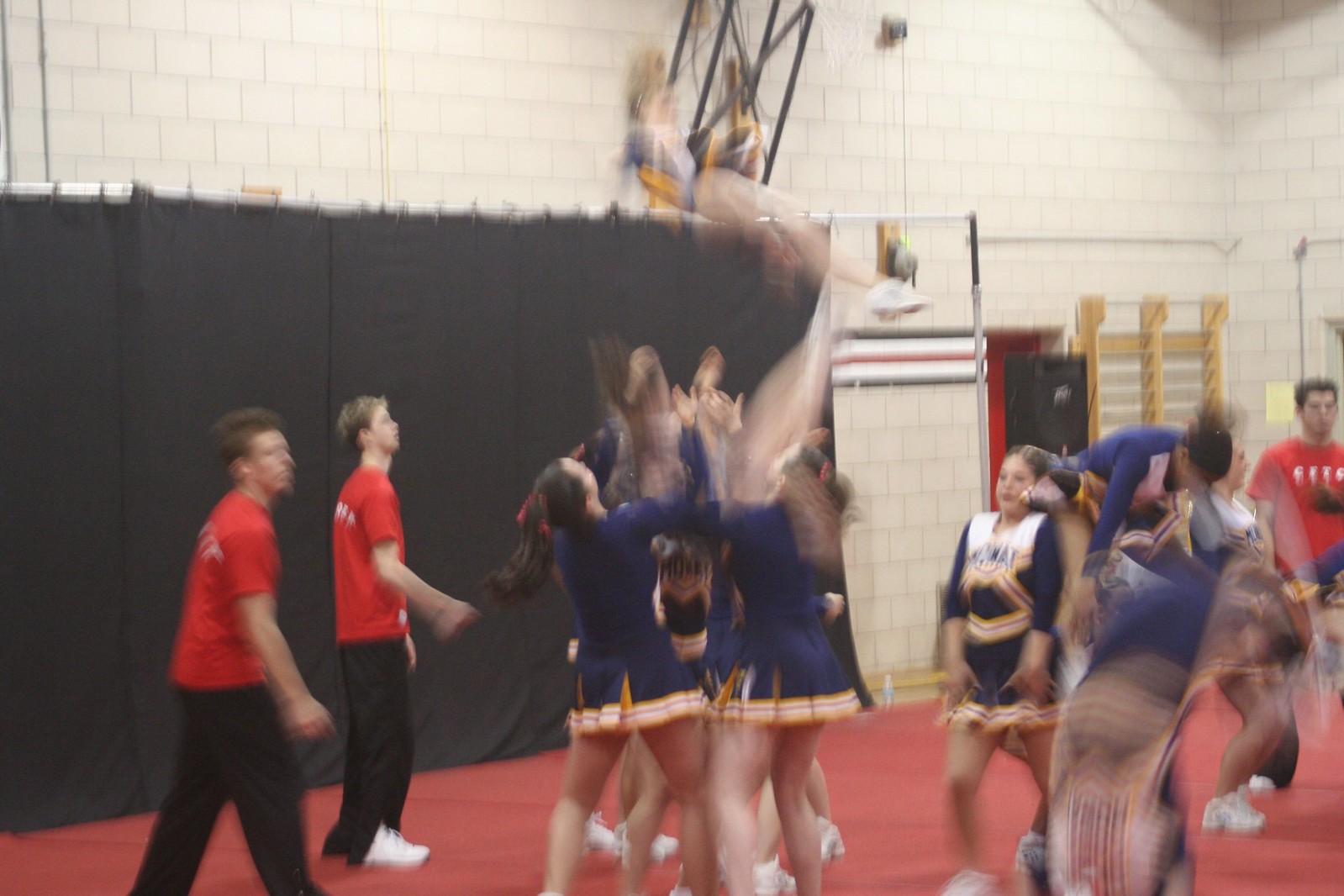This indoor photo captures a group of cheerleaders practicing in what appears to be a high school gymnasium. The image is slightly out of focus and the quality is not the best, making some details a bit fuzzy. The gym features white brick or cinder block walls and a red floor. In the background, a black curtain can be seen.

The cheerleaders, likely teenagers, wear striking blue costumes with orange and white accents. Their outfits feature orange at the bottom, a white section around the chest, and an orange shape with a hole under the chest, allowing the blue fabric to peek through. In the scene, one cheerleader is being thrown into the air, although her figure is blurred and hard to see clearly. Several other cheerleaders are on the ground, forming part of the practice routine.

Additionally, there are three boys in the image, acting as spotters. Two of them are positioned on the left-hand side and one on the right-hand side. The boys are dressed in red t-shirts and black pants, assisting the female cheerleaders with their formations.